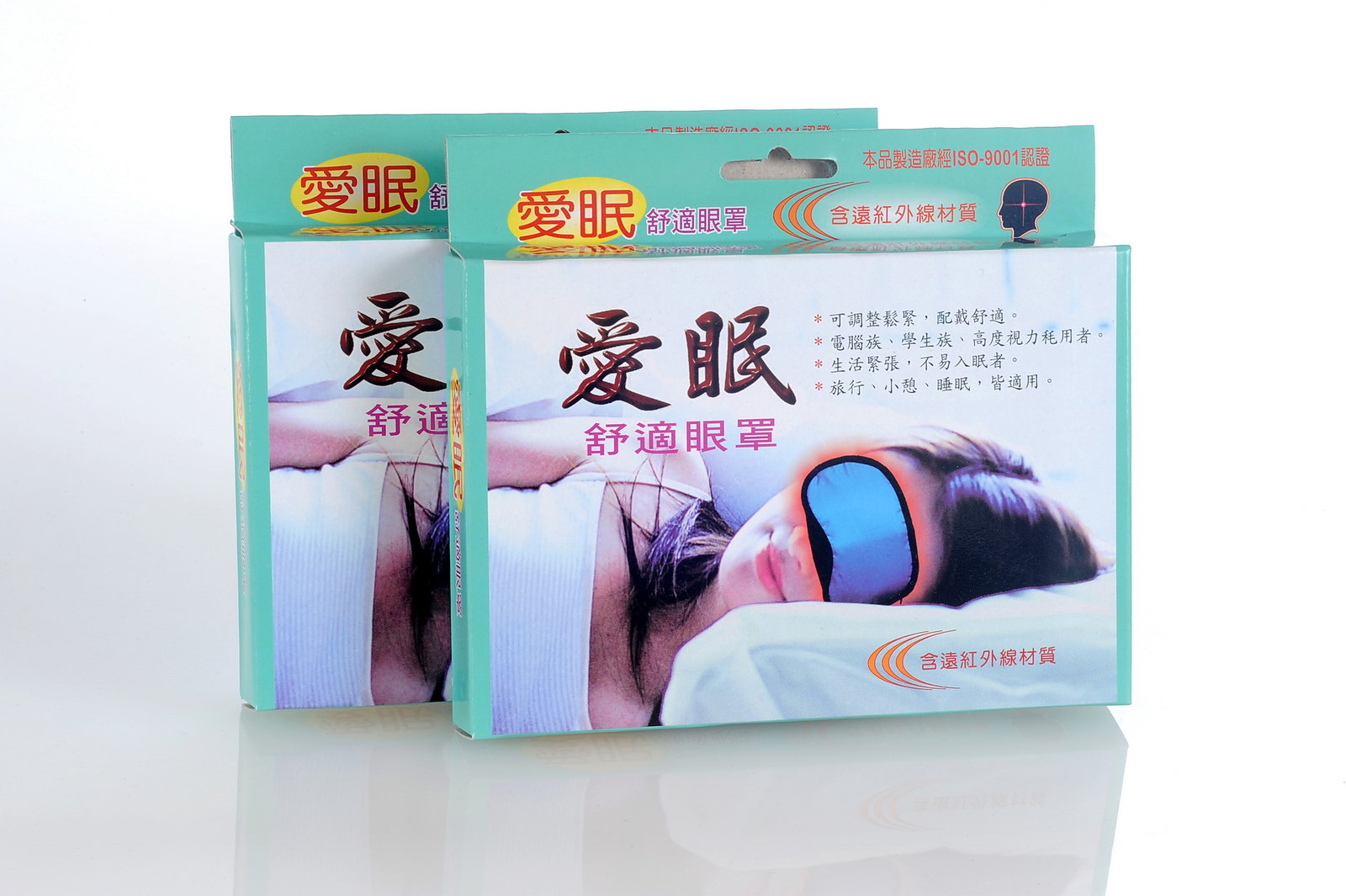This image depicts two turquoise blue boxes of sleep masks displayed on a white table. The box in the foreground is slightly overlapping the one behind it. Both boxes feature extensive Chinese writing. The primary visual on each box shows a young woman lying on her side with a contented smile, her head resting on a pillow. She has long brown hair cascading over her shoulders and she is wearing a white top. The woman is also adorned with a blue sleep mask that has a black border, and her serene expression is complemented by an illustrated orange aura emanating from the mask. The background is entirely white, reflecting a clean and minimalistic presentation.